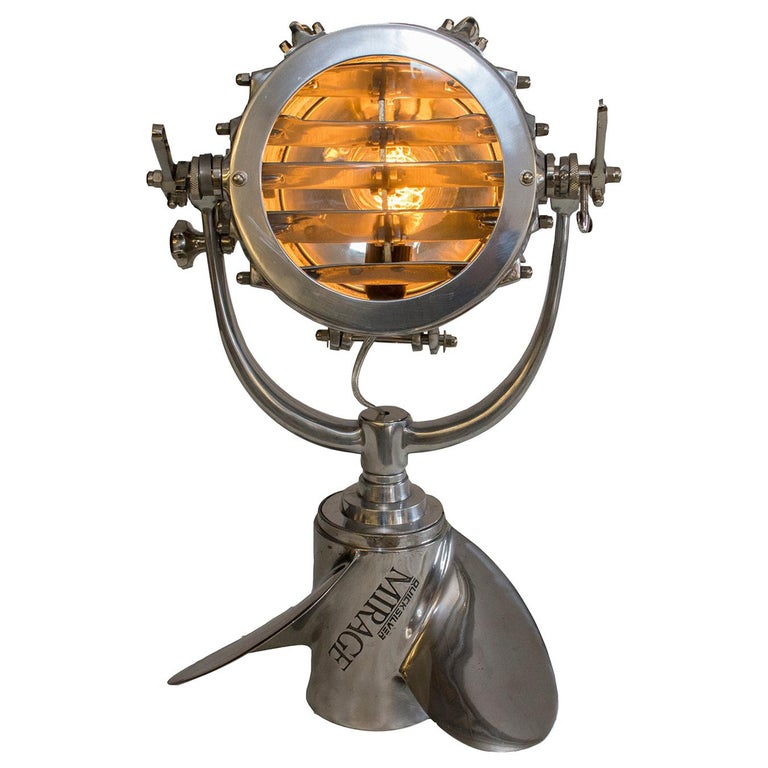This detailed photograph features a Quicksilver Mirage propeller, distinguished by its sleek silver finish. The propeller is dominated by a U-shaped metal piece extending upwards, indicative of its sturdy build. Centrally mounted is a circular component housing an amber-colored light bulb, casting a warm reflection inside the encasement. The design includes silver slats and several positional clamps, ensuring the central piece remains securely in place. Surrounding the central circle, a series of silver knobs are visible, adding to the industrial aesthetic. The bottom of the propeller catches and reflects light, highlighting its polished surface. The image is of excellent quality, offering a clear and sharp view of this intriguing, yet obscure piece of equipment. Notably, the photograph focuses solely on the propeller, with no other objects present in the frame.